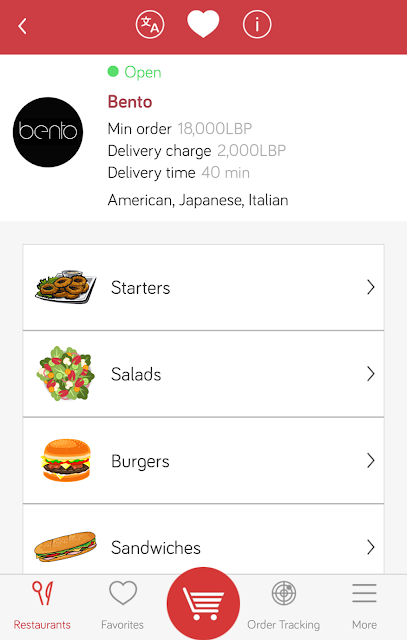This image features a webpage layout for a food delivery service. At the very top, there is a red banner stretching horizontally with a white heart icon, a white circle containing the letter "I," and another white circle with the letter "A." Below this banner, "open" is written in green with a small green dot beside it.

On the left side, a solid black circle presents the word "bento" in white text. Adjacent to this, "bento" is repeated in red writing, followed by a list in black text detailing "minimum order," "delivery charge," and "delivery time," along with the cuisine types - American, Japanese, and Italian.

The main section is segmented by categories: "starters," which includes an image of a white plate filled with golden onion rings; "salads," illustrated with a vibrant photo of fresh green leafy salad accented with red, orange, and white ingredients; "burgers," showing a burger layered with tomato, lettuce, and melted cheese; and "sandwiches," featuring an image of a long submarine sandwich.

On the right side, "restaurants" is written in bold red with icons of a spoon and knife above it. Beneath this, there is a white heart icon next to the word "favorites." A red circle containing a white shopping cart symbol and the phrase "order tracking" is also visible towards the right.